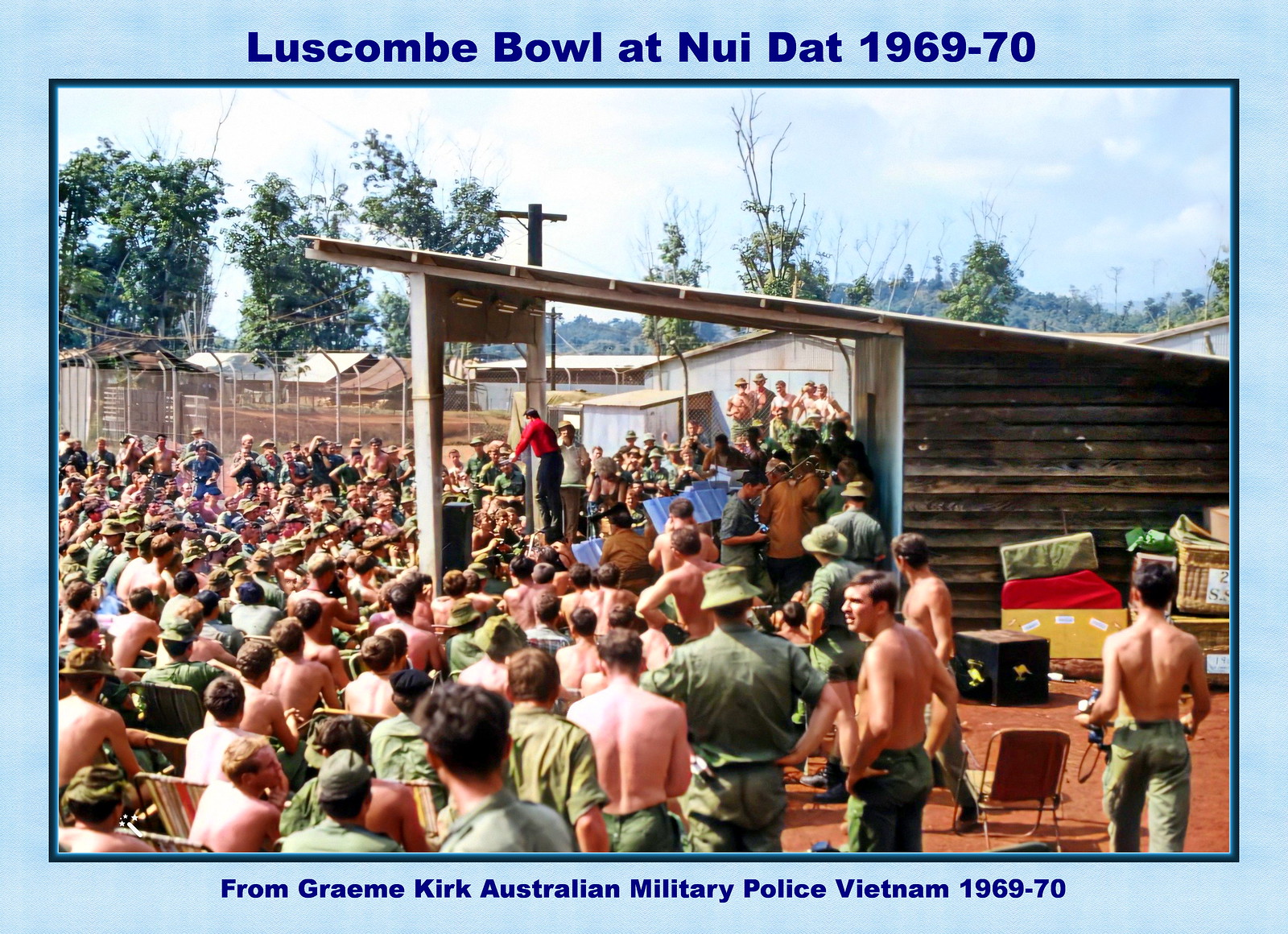The photo, outlined in blue, captures a historical moment labeled "Luscombe Bowl at Nui Dat, 1969-70." At the bottom, the caption reads, "From Graham Kirk, Australian Military Police, Vietnam 1969-70." The image features a large group of predominantly shirtless men, most likely military personnel, gathered during the Vietnam War. They are intently watching a performance on a stage, which is situated in front of a small pavilion or hut with an angled roof. The scene is bustling with several chairs and a man on the right holding a camera. In the background, a metal fence separates the main area from additional single-story huts, trees, and a distant mountain, reinforcing the setting's remote and rugged nature.